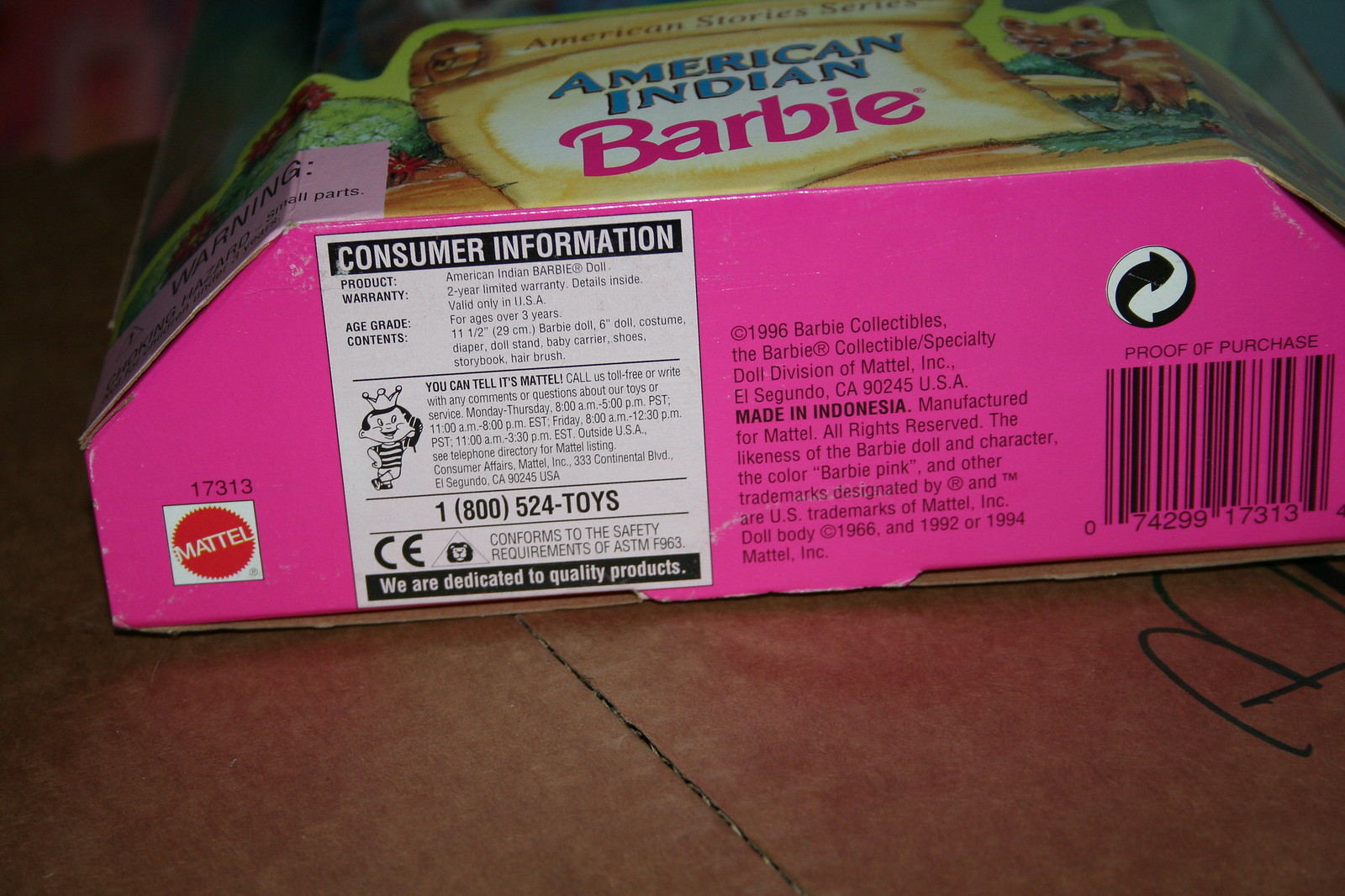This color snapshot photograph features an American Indian Barbie box prominently displayed on a table. The box is positioned so that its bottom edge runs diagonally from left to right across the center of the image. The bottom of the box is adorned with white text on a black background providing consumer information. To the left of this text is the iconic Mattel logo, presented within a red, sunburst-like circle, with the product number "17313" visible at the top.

Moving to the right of the consumer information, the words "Copyright 1996 Barbie Collectibles" are printed, along with manufacturing details. The lower part of the box includes a proof of purchase and a UPC symbol, all set against a vibrant pink background. 

At the top of the box, "American Indian Barbie" is written in prominent text, flanked by illustrative designs on both sides. The box itself rests on a piece of brown cardboard, which has the letter "B" hastily scribbled in black Sharpie marker in the lower right-hand corner. The overall presentation captures the classic aesthetic and intricate detailing of this collectible item.